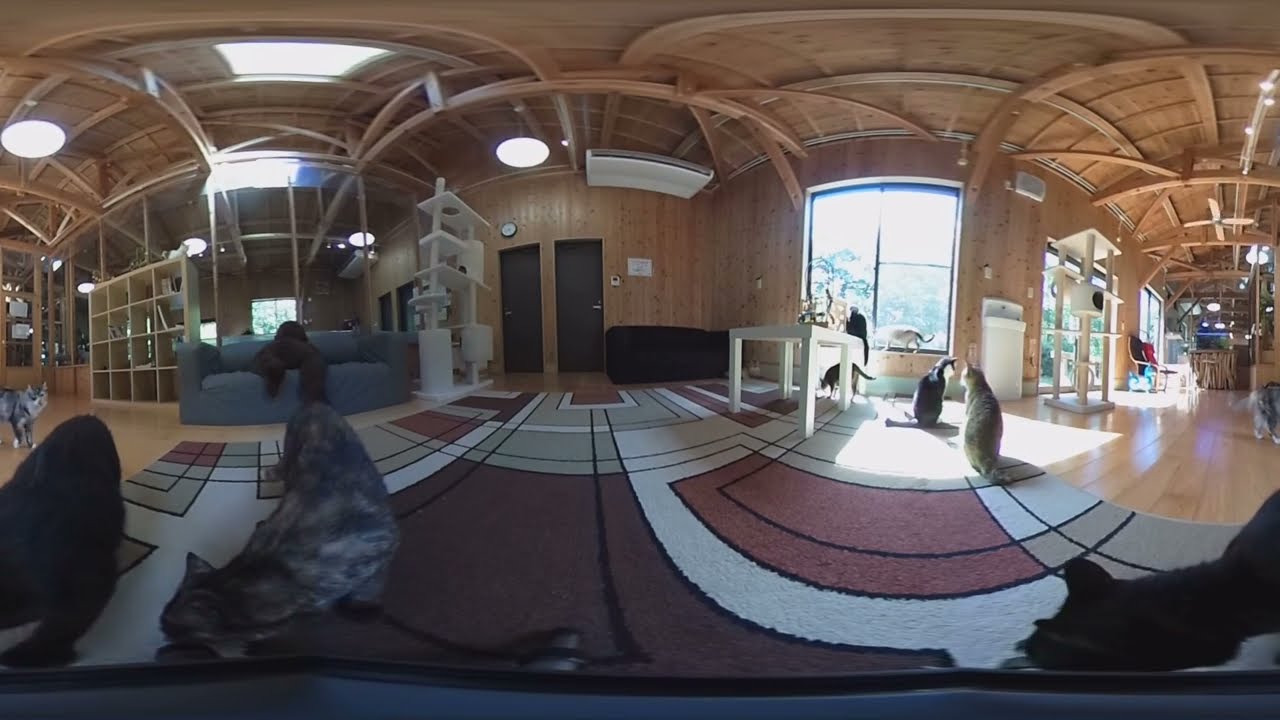The photograph captures the interior of a wooden-walled pet sanctuary, possibly inside a rustic cabin, bathed in natural daylight. Central to the image is a modern, art deco carpet with black, white, and red stripes laid across a hardwood floor. Cats of various colors, including a close-up black and gray calico, populate the space—some lounging in the sunlight streaming through a large picturesque window to the right. Adjacent to this window is a white table. The sanctuary features multiple cat-friendly amenities, such as a climbing wall and several doorways leading to more cat areas. To the left, a gray couch adds to the cozy ambience. The unfinished wooden roof and the array of colors—black, brown, white, blue, green, pink, tan, and gray—complete this warm and lively setting.